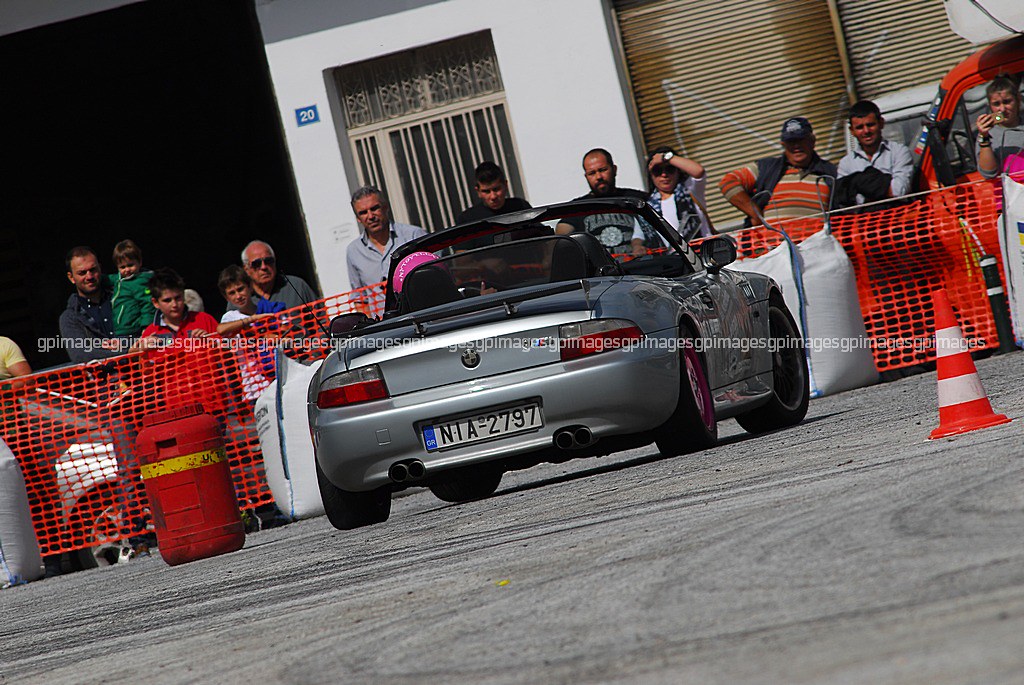In an outdoor setting, a luxurious car takes center stage with a driver donning a bright pink helmet seated inside. The car's license plate reads "NIA 2797." A group of onlookers gathers behind an orange plastic fence, closely inspecting the vehicle. On the right, an orange and white traffic cone is positioned on a surface that appears to be made of gravel or dirt. In the background, a white building marked with the number "20" and featuring a blue box looms over the scene. The sun, descending from behind the camera, causes the spectators to shield their eyes or wear sunglasses. The image also contains copyright text in a stylized font overlaying the scene.